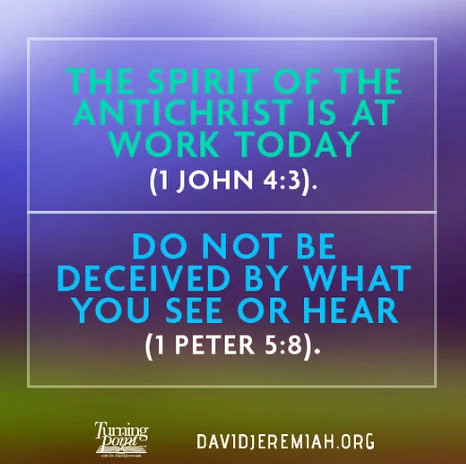The image is an advertisement for a religious service, designed for social media platforms like Instagram. It features a gradient backdrop transitioning from purple to green with a soft, blurry effect. At the top of the graphic, green text reads, "The spirit of the Antichrist is at work today," followed by the attribution in white text, "1 John 4:3." Below it, in blue text, the image reads, "Do not be deceived by what you see or hear," with the white attribution, "1 Peter 5:8." At the bottom, the logo for "Turning Point" is positioned on the left side, while on the right side, the URL "DavidJeremiah.org" is prominently displayed.